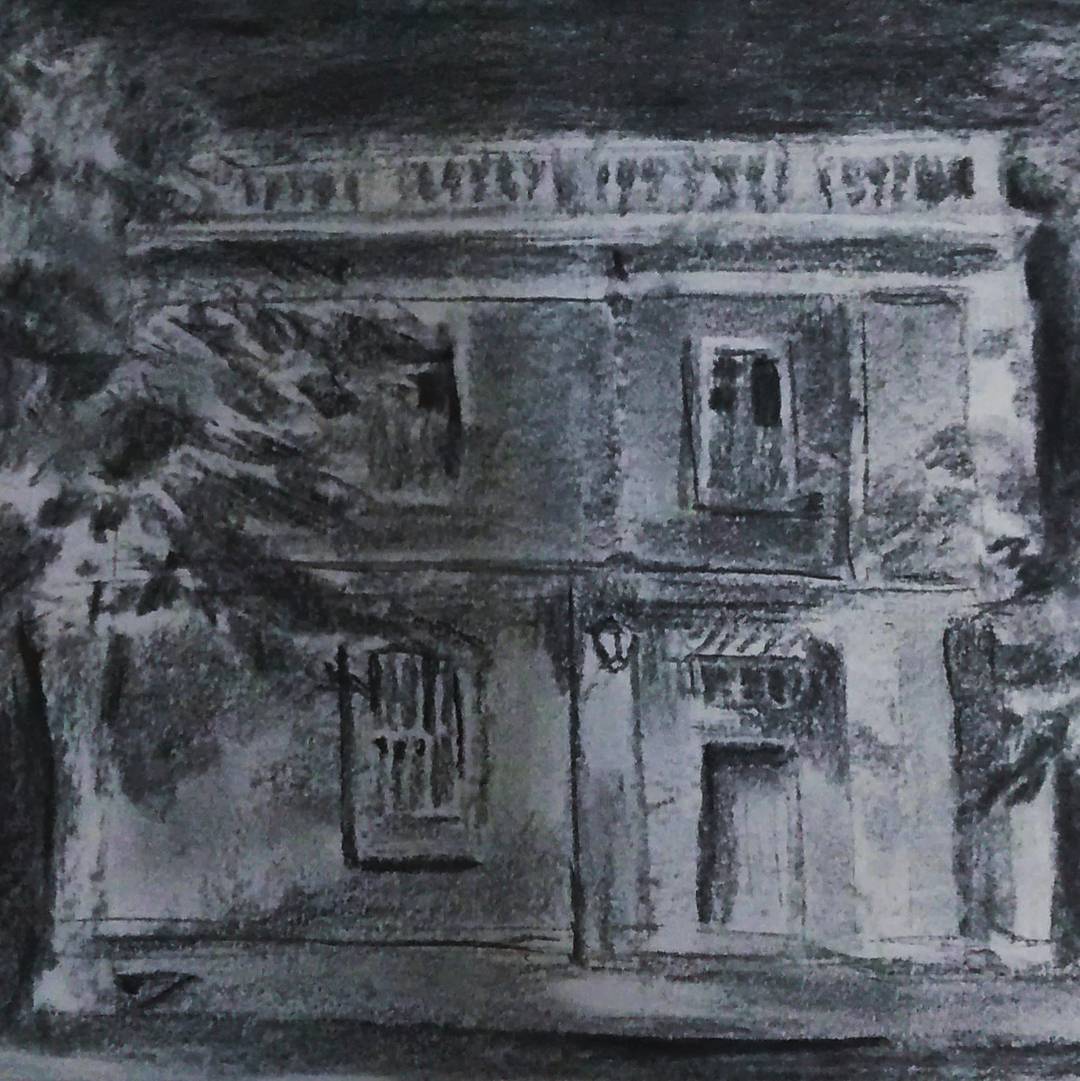This is a highly detailed black-and-white sketch of a two-story building. The front of the building features a minimalist door located at the bottom right-hand side, with a dark outline making it hard to discern fine details. Above the door, on the second floor, there's a rectangular window, black at the top and white at the bottom. Directly opposite, on the building's left side, is another window partially obscured by what appears to be a tree with leaves blowing to the right. Below this upper window, there is a second window, also slightly covered by leaves. Additional architectural elements include a possible light post diagonally above the door and a dark, indistinguishable feature that might be a balcony or roof element. The scene is set against a predominantly dark, nighttime background, further emphasizing the black shading of both the building and the tree. A sidewalk extends across the front of the building, grounding the scene in a more lifelike setting.